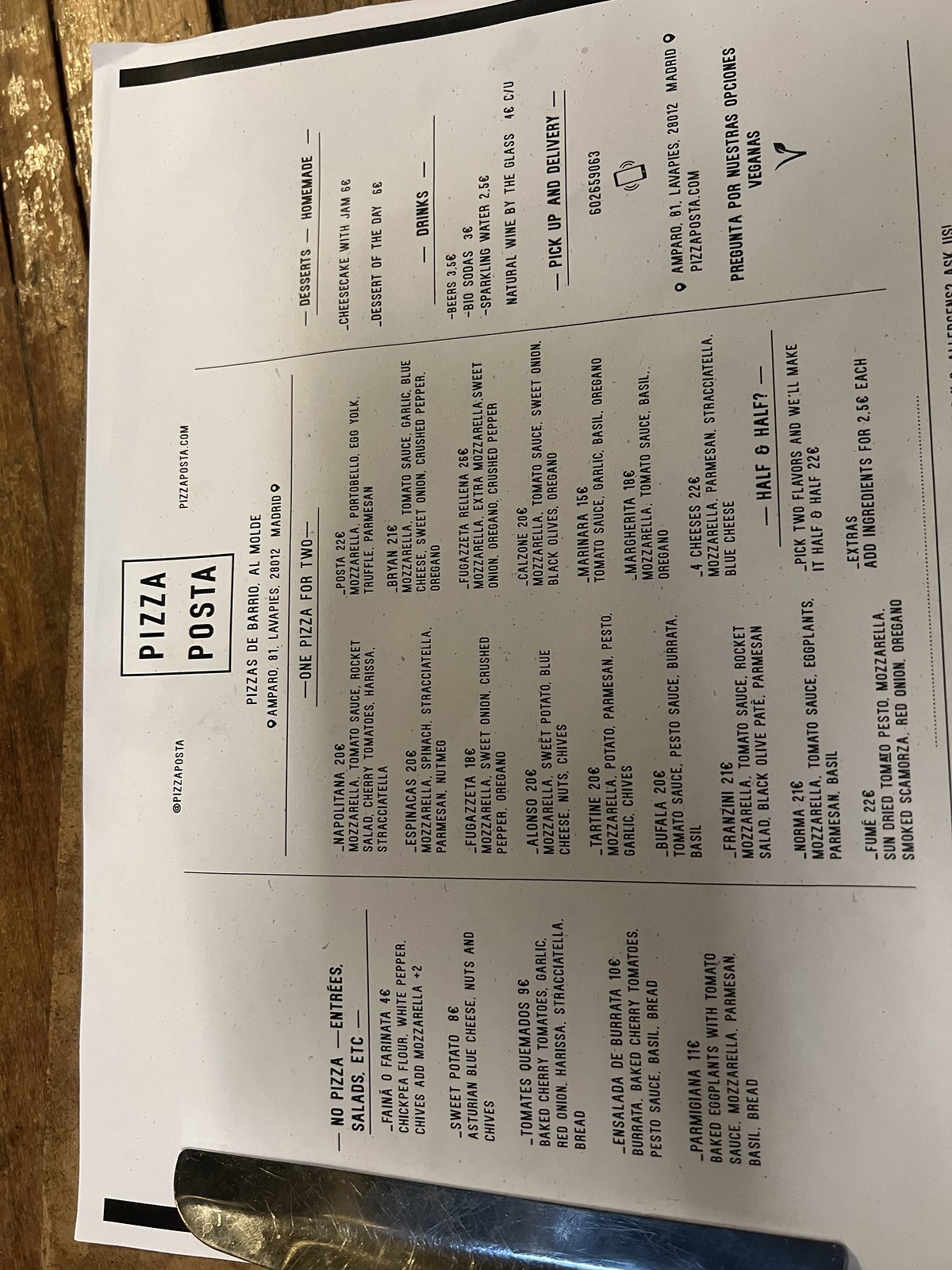This image features a metallic piece of paper clipped to a wooden surface with a long metal clip. The paper itself is organized into three sections by two vertical lines. At the top center, there is a outlined square containing the text "Pizza Posta." Beneath this header is the address of the establishment, followed by parts of the menu.

On the left side of the paper are the menu categories "Pizza," "Entrees," and "Salads," along with their respective options listed underneath. The middle section lists "One Pizza for Two" with available choices below, and "Half and Half" with two options provided beneath it. The right side of the paper displays "Desserts," denoted as "Homemade," along with two listed options. Additionally, it features "Drinks" with several choices and "Pickup and Delivery" accompanied by a phone number and a cell phone symbol. There is also more text written underneath the contact information.